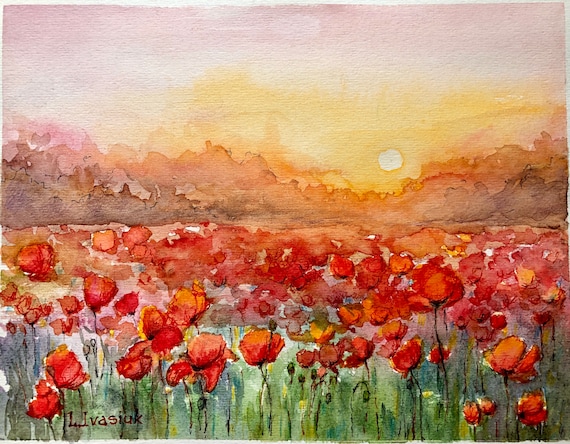This watercolor painting, signed by L. I. Vasyuk in the lower left corner, vividly captures a sprawling field of red flowers, potentially tulips or poppies. The flowers, accented with hints of orange, dominate the foreground with well-defined petals and green stems, transitioning into a blur of red hues towards the horizon. In the background, a range of brownish-gray hills or mountains rises, framed by a sky painted in gradients of grayish purple to soft, glowing oranges, and pinks. Above the hills, a radiant yellow sun, flanked by a halo of intensifying orange, suggests either a sunrise or sunset. Darker purple clouds float near the sun, adding depth and contrast to the serene landscape.